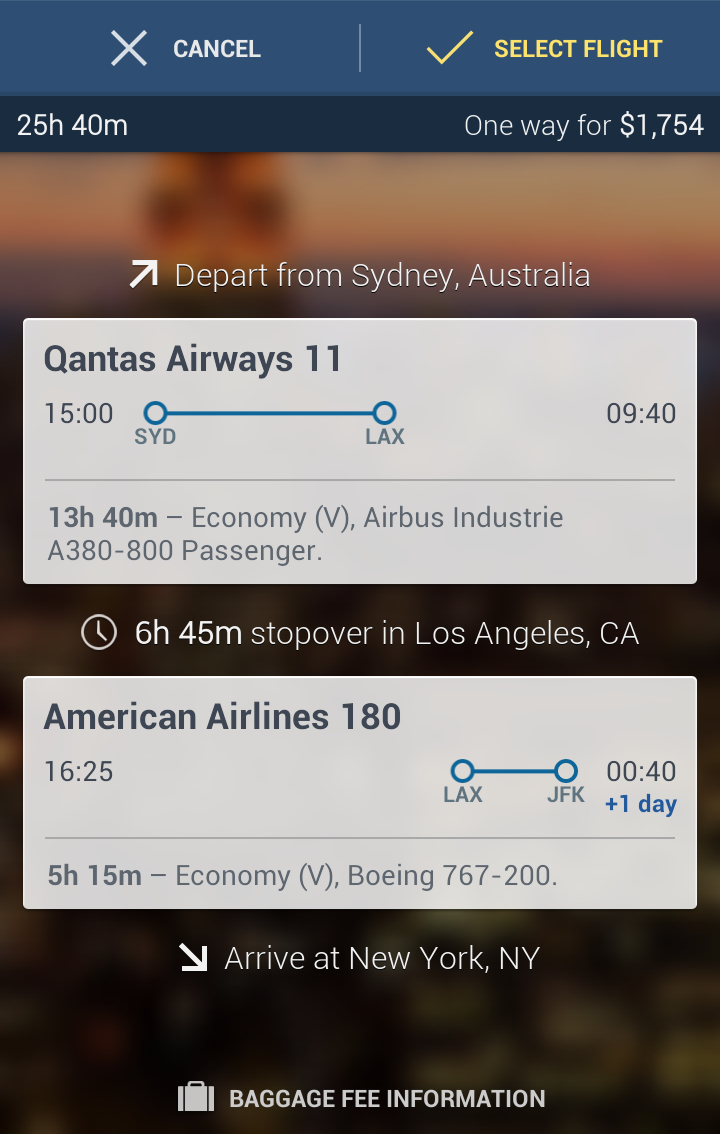In this screenshot capturing information related to baggage for Qantas and American Airlines, the page is organized with several distinct visual elements. At the top, there is a blue banner featuring a noticeable "X" icon labeled "cancel." Next to it, a vertical line leads to a yellow checkmark icon saying "select flight." Below this, a black bar displays crucial travel details: "25 hours 40 minutes one way for $1,754."

The background of the image has an orange to orangey-tan hue, but it is blurred and not clearly visible. An upward-pointing arrow directs attention to the upper right-hand corner, where it mentions "depart from Sydney, Australia."

A white box stands out prominently, showcasing "Qantas Airways 11" in bold letters. Adjacent to it, the timing "15:15" is displayed, following the 24-hour time format. A connecting blue circle labeled "SYD" (Sydney) links via a line to an open blue circle marked "LAX" (Los Angeles), along with the time "09:40."

A gray horizontal line separates this section from additional flight details, stating "13 hours 40 minutes - economy (V), Airbus A380-800 passenger."